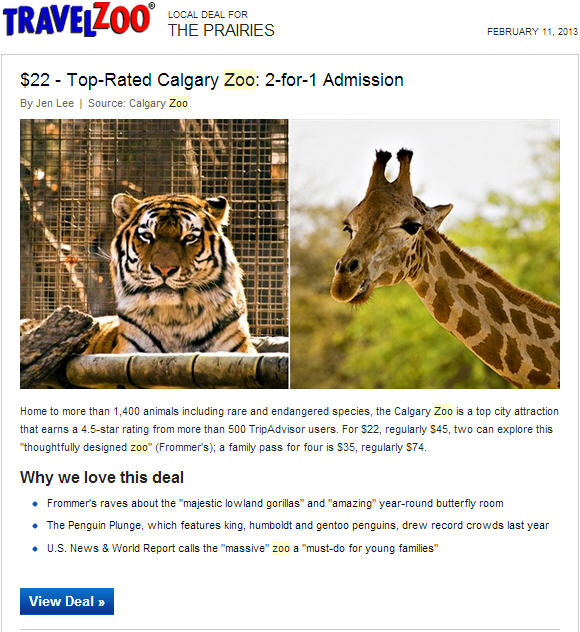In this image set against a white background, we see a screenshot of a web page. In the upper left corner, the website company "Travel Zoo" is prominently displayed, with "Travel" in bold blue print and "Zoo" in bold red print. To the right of the logo, in black print, it says "Local Deal for the Prairies." In the upper right corner, the date "February 11th, 2013" is displayed.

Beneath this header, there is a gray-lined bordered white box. In the top left corner of the box, a deal is highlighted: "$22 Top-Rated Calgary Zoo Two-for-One Admission" by Jen Lee. The source of the information is noted as "Calgary Zoo." Below this information are two side-by-side photographs. 

The photo on the left features a tiger in a zoo environment, looking forward with a focused gaze. The right photo showcases a giraffe, its long neck emerging from the lower right side of the image. Behind the giraffe, a backdrop of greenery and sky is visible, enhancing the natural charm of the scene.